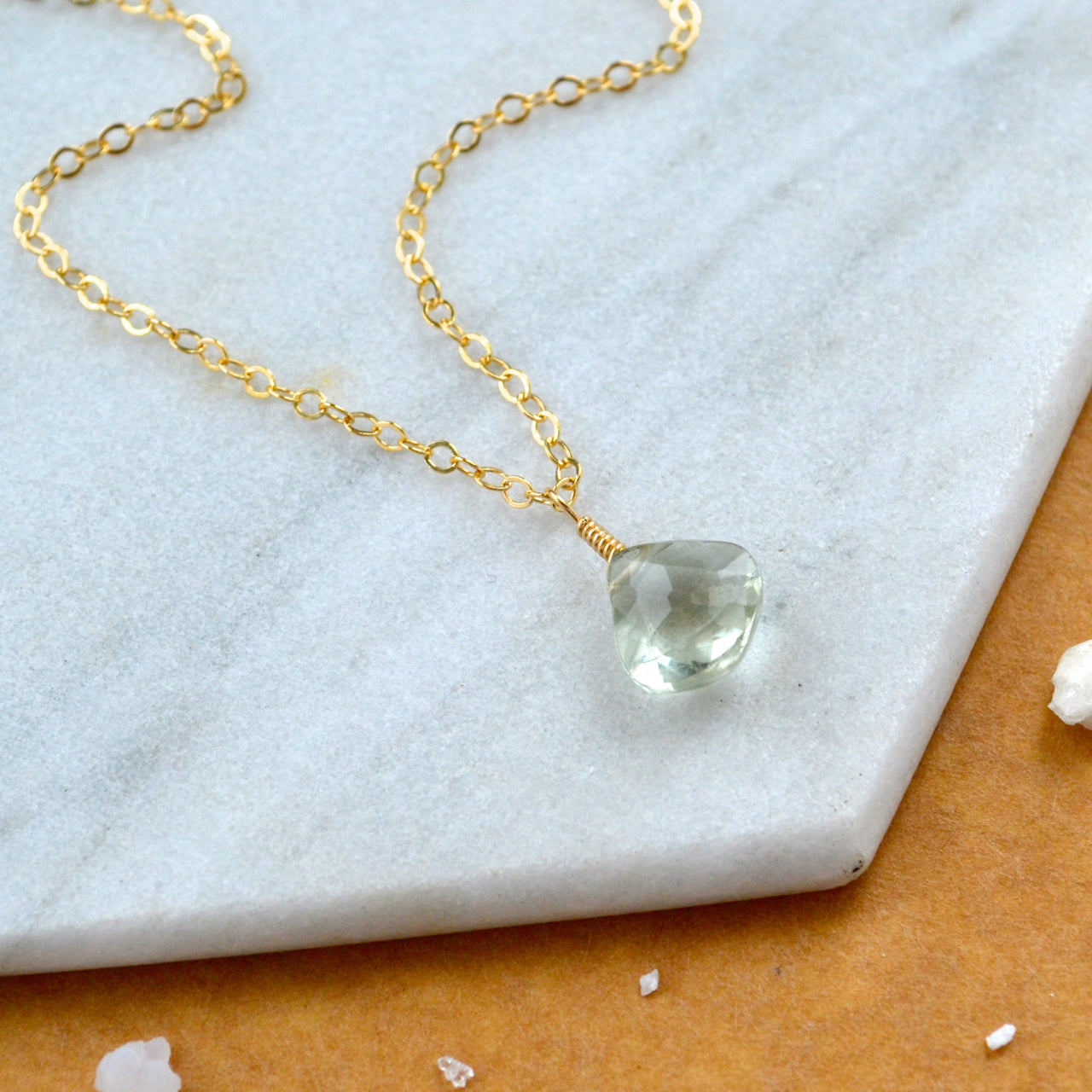The photograph showcases a striking necklace resting on a gray and white marble surface that is, in turn, placed on a brownish flat surface. The marble surface features an obtuse-angled corner near the bottom right, highlighting its unique geometry. A stunning teardrop-shaped crystal, resembling a large, clear diamond, elegantly hangs from the golden chain of the necklace, which extends upward across the center of the image. Scattered around the marble are small white shards or chips, possibly pieces of rock or mineral, visible particularly in the right center and lower left corners of the brown background. The overall composition exudes a sense of refined luxury, combining the gleam of the crystal with the subtle textures of the marble and the contrasting brown surface.